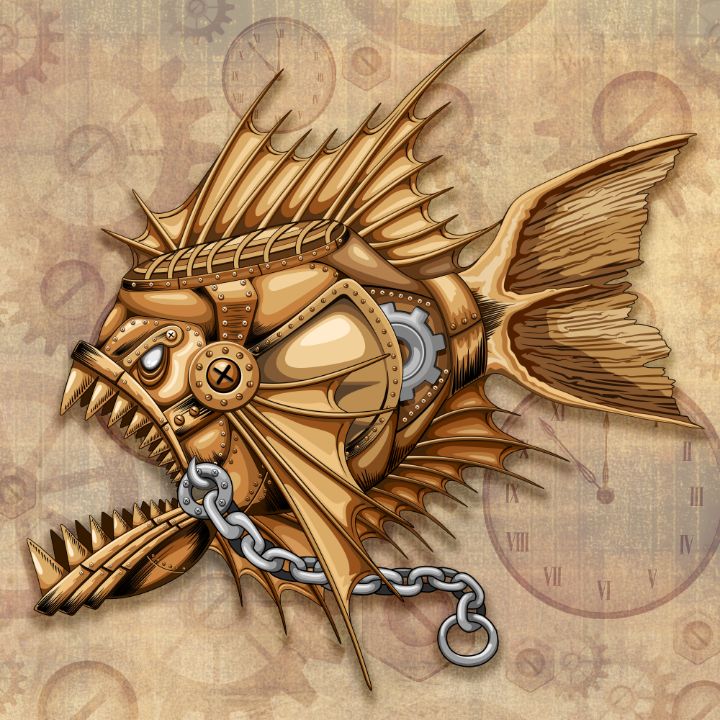This digital illustration depicts a mechanical, gold-colored piranha-like fish. The fish is facing left with its mouth wide open, revealing long, sharp teeth along the edges. A thick, silver chain is hooked in the center of its mouth, extending rightward before hanging down. The fish's eye is white, and directly behind it is a circle resembling a screw with an X in it. Above this area, a flat portion is adorned with brown lines. The fish's top fin is pointed and forked, with two points extending to the upper left and the remaining points to the right. Its jagged tail fin is wide, and both fins and tail exhibit a metal-plated, gold-armored appearance. A gray gear with notched edges is prominently embedded in the middle of the fish. The illustration's background consists of a tan backdrop with light brown and light purple silhouettes of variously sized gears and analog clocks, adding a steampunk aesthetic to the overall image.